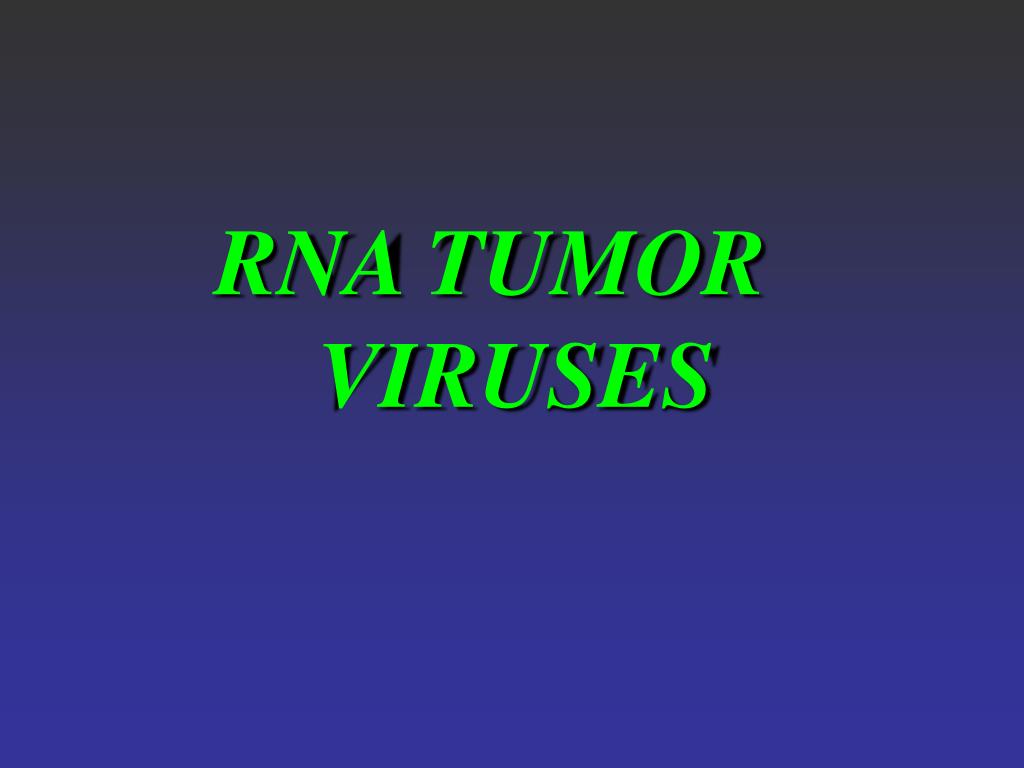The image is a PowerPoint slide with a gradient background that transitions from a very dark, almost black at the top, to a royal blue at the bottom. Centered in the upper half of the slide are two lines of text reading "RNA TUMOR" on the first line and "VIRUSES" on the second line, both written in neon green, all capital letters. The text features an italicized font with a subtle black shadow effect, enhancing the visibility of the letters. There are no other objects or text on the slide.